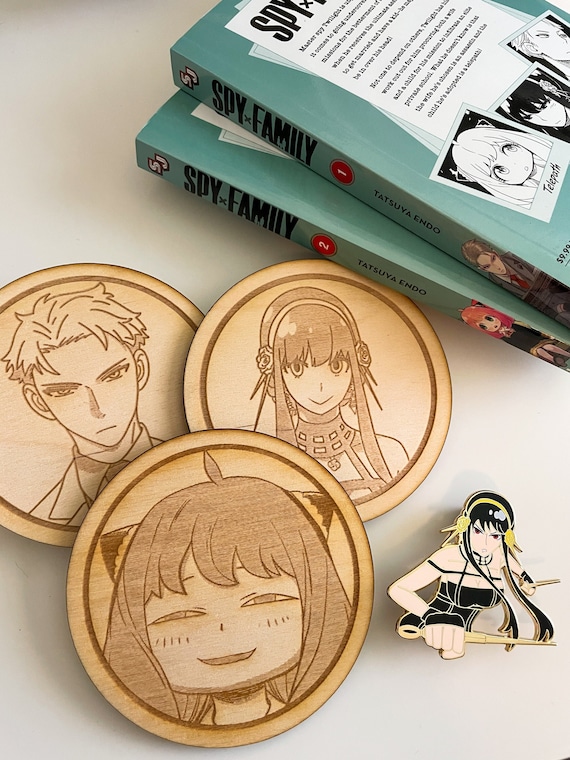The image depicts three round, coin-shaped wooden discs positioned against a cream-colored background. Each disc features detailed laser-etched engravings of anime characters. The front disc showcases a young girl with a bob haircut, bangs, cat ears, and tiny eyes paired with long fangs. Behind her to the left is a disc with a male character, identifiable by his short, spiky blond hair and a sharp expression. The third disc, positioned between the other two, features a female character who wears her hair long with a headband and earphones, including long side pieces.

To the right of these discs, there is a smaller, colored wooden cutout of the same female character in a black dress, holding a weapon in each hand. This cutout is propped up against two stacked books with green covers, identified as volumes one and two of the manga series "Spy Family" by Tatsuya Endo. The book covers display imagery and text related to the series, including small black and white portraits labeled with roles like "telepath."